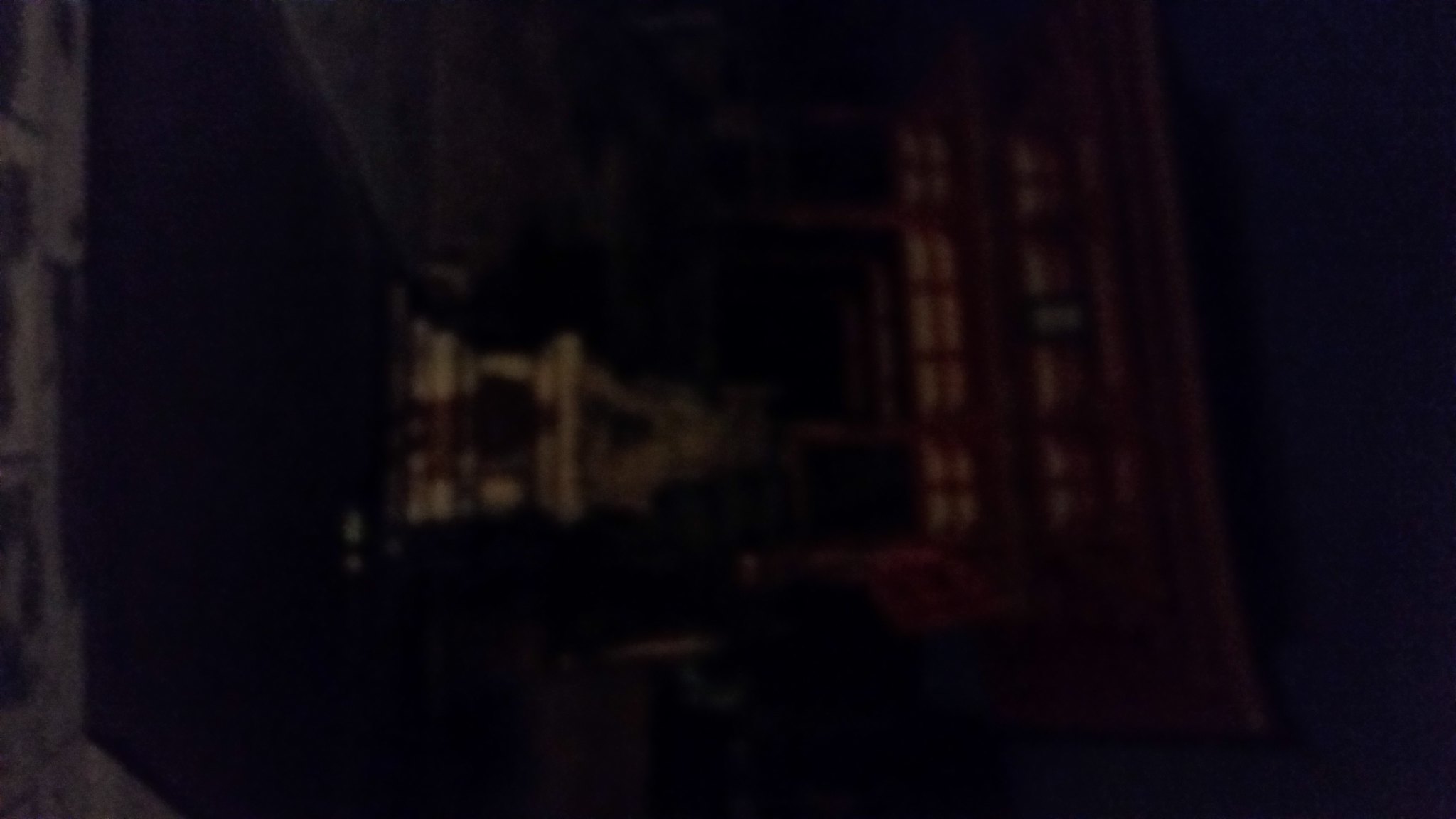This image appears to be a poorly lit, low-quality photograph, possibly taken at night or in the late evening, making it challenging to discern details. The photo seems to be captured outdoors, possibly at an Asian shrine, characterized by dim lighting which contributes to its grainy and blurry quality. The orientation of the image is off, likely taken in portrait mode but displayed on its side.

In the central part of the image, an outline resembling a red shrine with traditional Asian architectural features can be vaguely seen. There appears to be a white section that might be a table or shelf, with a dark spot that could be a stool or chair. Further, there is a suggestion of a statue amidst the shadows, and what looks like a purple carpet on the ground. Towards the building's outline, which seems tall with several stories, lights in the windows can barely be made out. On the left side of the image, there's a white post or structure, although its exact nature is indistinct. To the right, there appears to be a brown door or window linked to a storefront with a sign that has black and white writing. A checkered shadow pattern is observed above it, adding to the overall obscurity of this enigmatic scene.